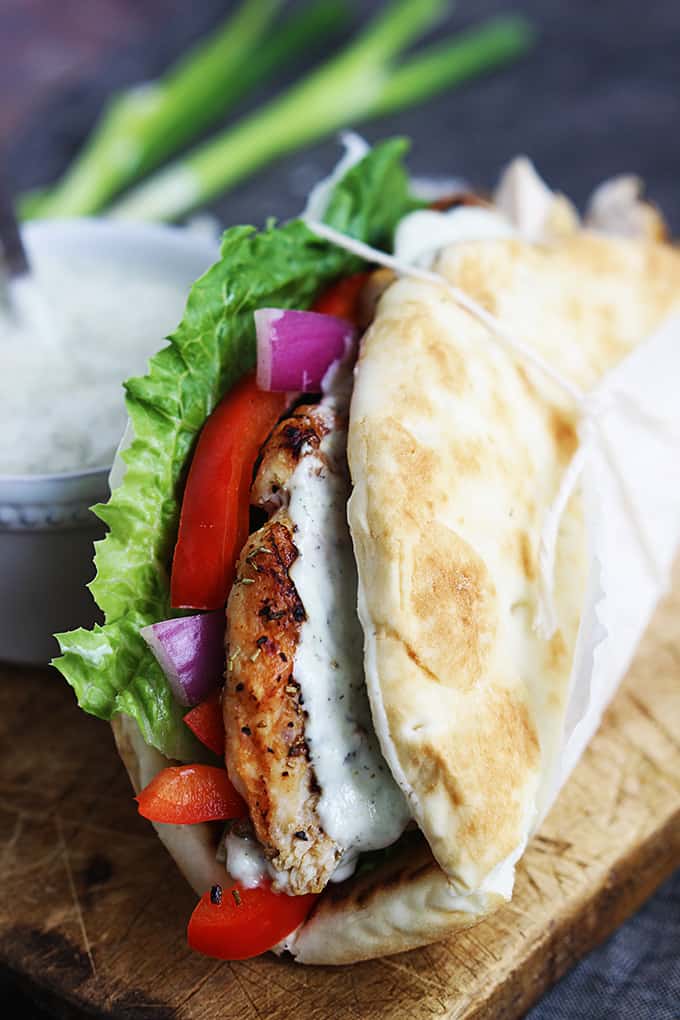Here is a detailed and cleaned-up descriptive caption:

"A mouthwatering Greek grilled chicken sandwich is showcased in this image. The sandwich features a thick, freshly baked pita bread stuffed with a crisp romaine lettuce leaf, juicy slices of tomato, vibrant red bell pepper strips, and slices of pungent purple onion. Nestled within the sandwich is a succulent, well-seasoned grilled chicken breast generously drizzled with creamy tzatziki sauce, a yogurt-based dressing infused with garlic and herbs. Beside the sandwich, a small container with a serving spoon handle peeking out holds extra sauce for added flavor. Two sprigs of fresh greenery, possibly scallions or lettuce leaves, rest next to the container. All these elements sit on a rustic wooden surface, marked with character-rich slice marks, suggesting it could be a well-used table or cutting board, adding to the authentic and homely appeal of the scene."